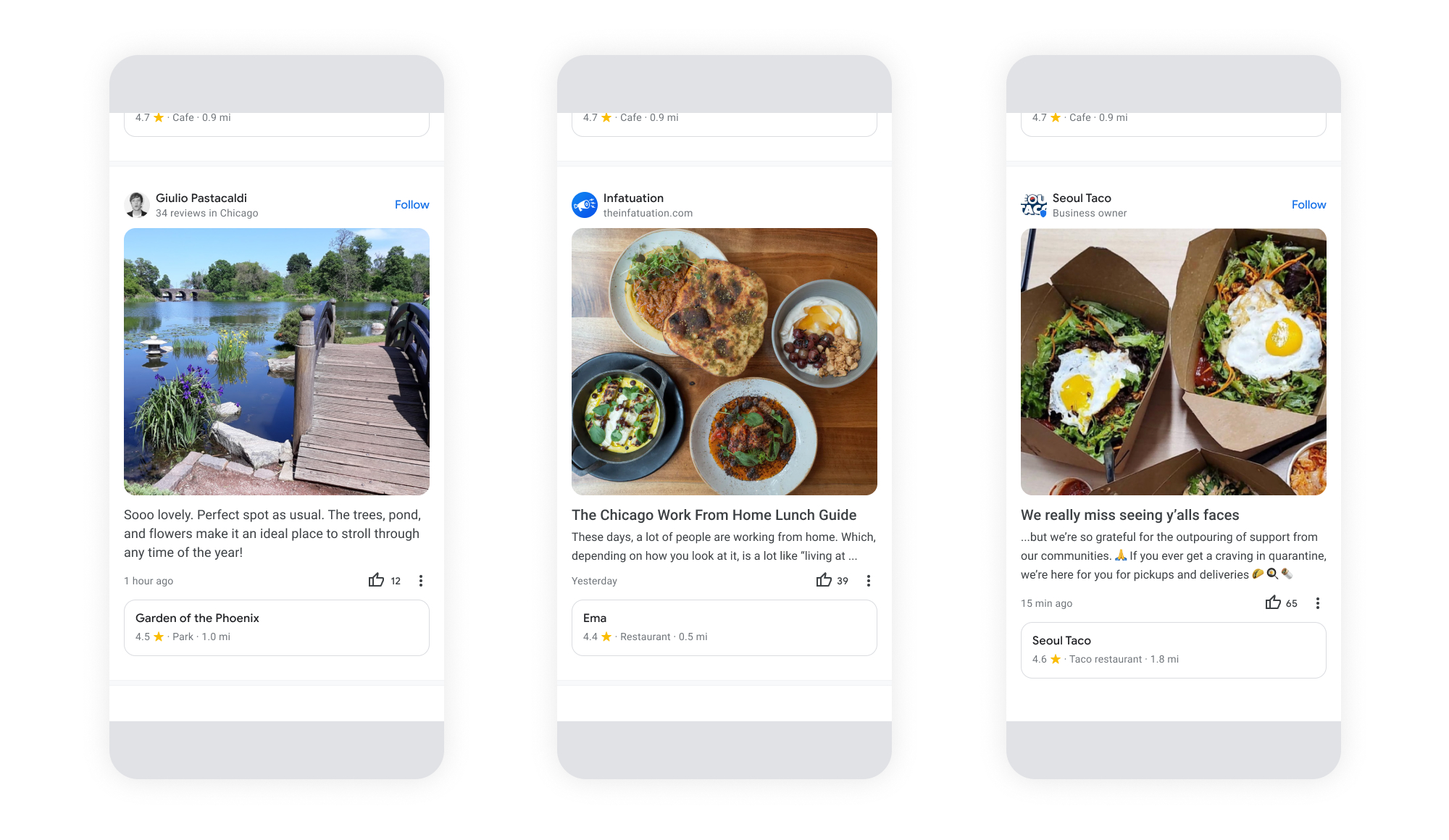The image captures three distinct cell phone screenshots of various search results, each reflecting different content. At the top, the header reads "Gulio Pastacaldi," displaying 34 reviews in Chicago, with an option to follow them.

The first screenshot showcases a picturesque scene of a serene pond or lake, adorned with a charming wooden bridge and surrounded by blooming flowers. The caption reads: "So lovely, perfect spot as usual. The trees, pond, and flowers make it an ideal place to stroll through any time of the year." This post was made an hour ago and has garnered 12 likes.

The second screenshot features an appetizing array of four different entrees, emphasizing the delightful experience of a work-from-home lunch. The accompanying text is from "The Infatuation" on theinfatuation.com, titled "The Chicago Work From Home Lunch Guide." The description highlights the increasing trend of working from home and its impact on daily life. Posted yesterday, this entry has received 39 likes.

The third screenshot depicts meals that prominently include eggs and salads from "CO Taco." The message conveys a sense of community support and gratitude during times of quarantine. It reads: "We really miss seeing y'all's faces, but we're so grateful for the outpouring of support from our communities. If you ever get a craving in quarantine, we're here for your pickup and deliveries."

Each screenshot captures a distinct aspect of life, from tranquil nature spots to culinary delights, all unified by a sense of community and shared experiences.